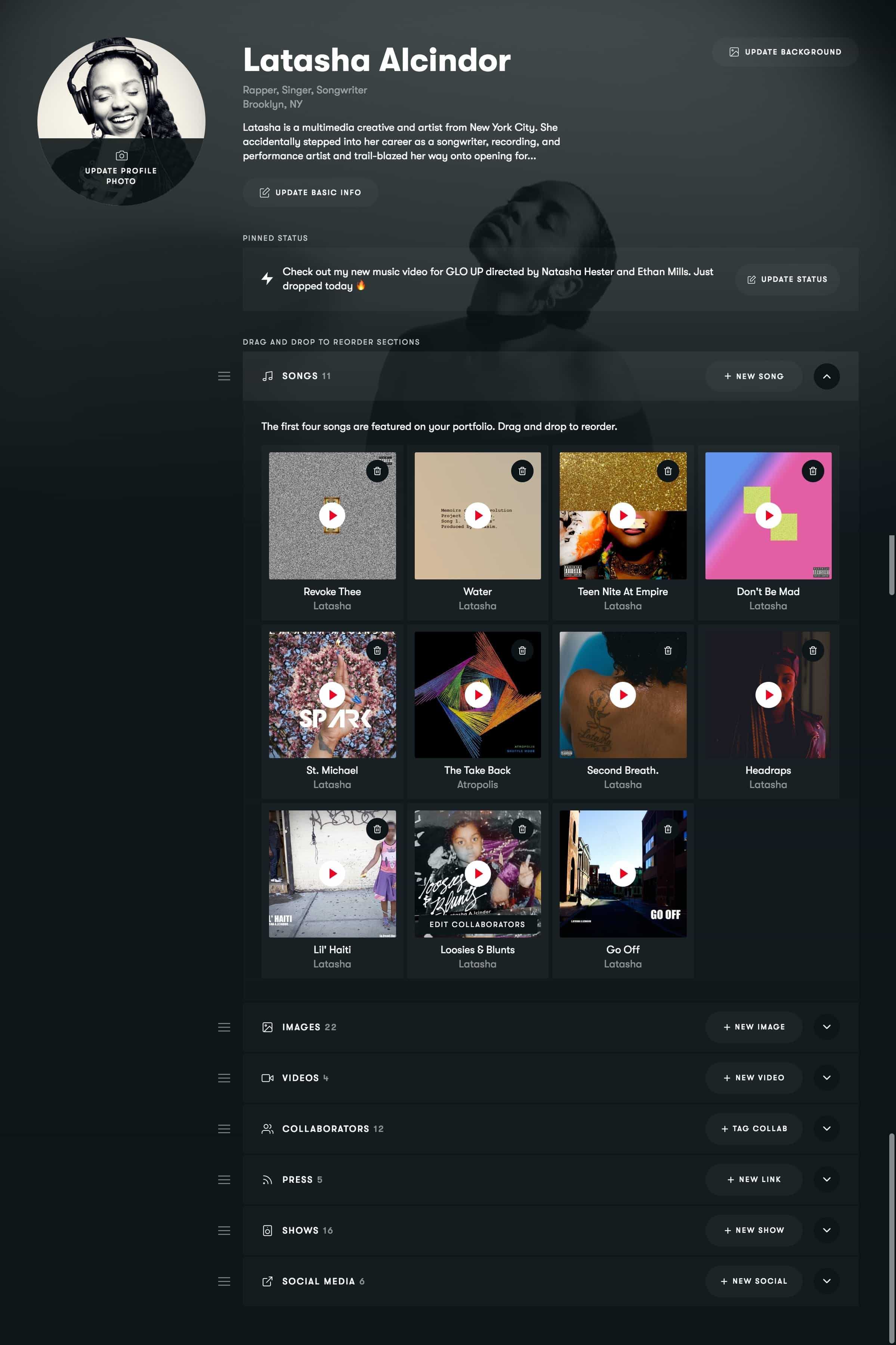A screen capture from a mobile digital device displays the profile page of artist Latasha Alcindor. The screen has a sophisticated deep purple-gray background. Prominently on the left, there is a monochromatic, round image of a woman wearing headphones. Adjacent to this, on the right, the artist's name, "Latasha Alcindor," is clearly written in bold white letters. Beneath her name, smaller white text provides additional details, although they are barely legible.

At the center of the screen, a grid of playlists is neatly arranged in three rows and four columns. Each playlist features a distinctive image of people and places, accompanied by a small, round play button in white and red. Further down on the screen, there are additional rows of information displayed in white text, though the font is quite small, making it challenging to read. The overall layout is well-organized, showcasing the artist's online presence effectively.